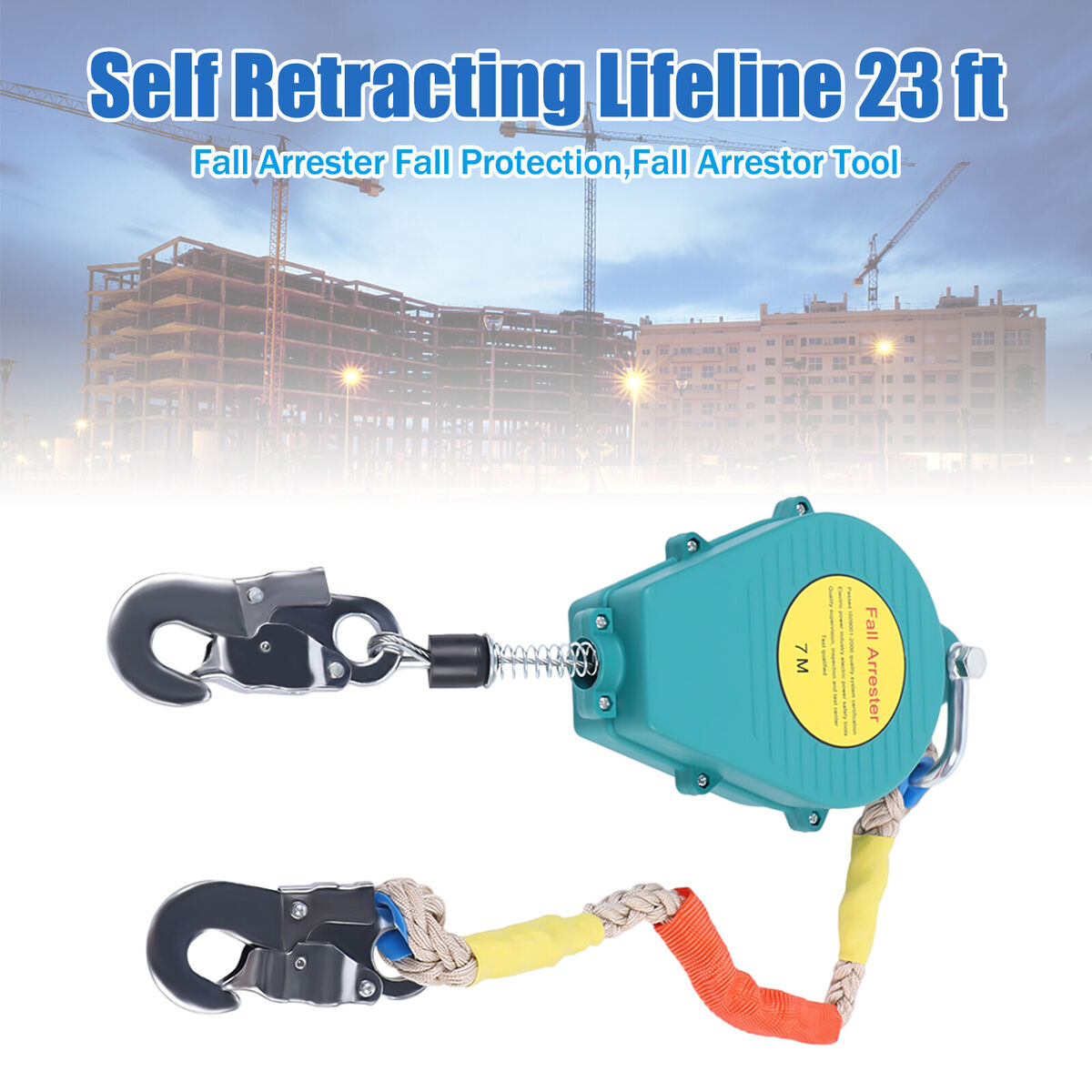This advertisement image prominently features a "Self-Retracting Lifeline, 23 feet" fall arrestor tool. The text at the top, displayed in bold blue with a white border, emphasizes its purpose as a fall protection device. Below the text, there is an image of a six-story building under construction, characterized by exposed iron framing and cranes, set against a cloudy sky. The structure is in its early stages, allowing a glimpse into its skeletal interior. At the bottom, the product itself is showcased against a white background. The device resembles the top of a hot air balloon turned sideways, featuring a blue case with visible screws and a yellow label stating "Fall Arrester 7M." A sturdy cable with yellow and orange portions emerges from the right side, ending in a large silver metal clasp, while a metal hook attached to a spring extends from the left side. The overall design highlights durability and safety, essential for fall protection in construction environments.